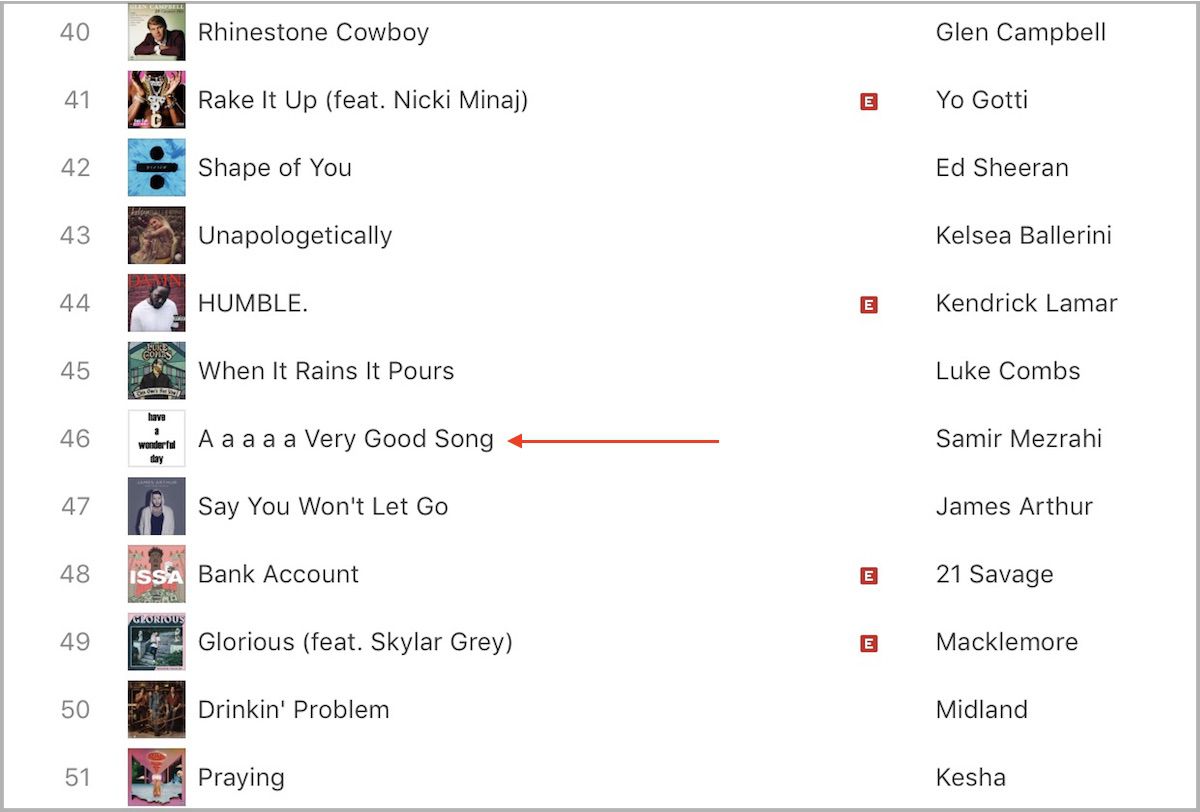This is a detailed screenshot of a music streaming or collection listing website, displaying a segment of a song list featuring positions 40 through 51. The list includes a variety of songs and artists, presented as follows:

- **40.** "Rhinestone Cowboy" by Glen Campbell
- **41.** "Break It Up" featuring Nicki Minaj by Yo Gotti
- **42.** "Shape of You" by Ed Sheeran
- **43.** "Unapologetically" by Kelsea Ballerini
- **44.** "HUMBLE." by Kendrick Lamar
- **45.** "When It Rains It Pours" by Luke Combs
- **46.** "A-A-A-A Very Good Song" by Samir Mazreha
- **47.** "Say You Won't Let Go" by James Arthur
- **48.** "Bank Account" by 21 Savage
- **49.** "Glorious" featuring Skylar Grey by Macklemore
- **50.** "Drinking Problem" by Midland
- **51.** "Praying" by Kesha

Highlighted within this section, "A-A-A-A Very Good Song" (number 46) is marked distinctly with a prominent red arrow, signifying its special status on the list. Additionally, several songs are tagged with a red box containing a white letter "E," indicating explicit content: "Break It Up" (41), "HUMBLE." (44), "Bank Account" (48), and "Glorious" (49).